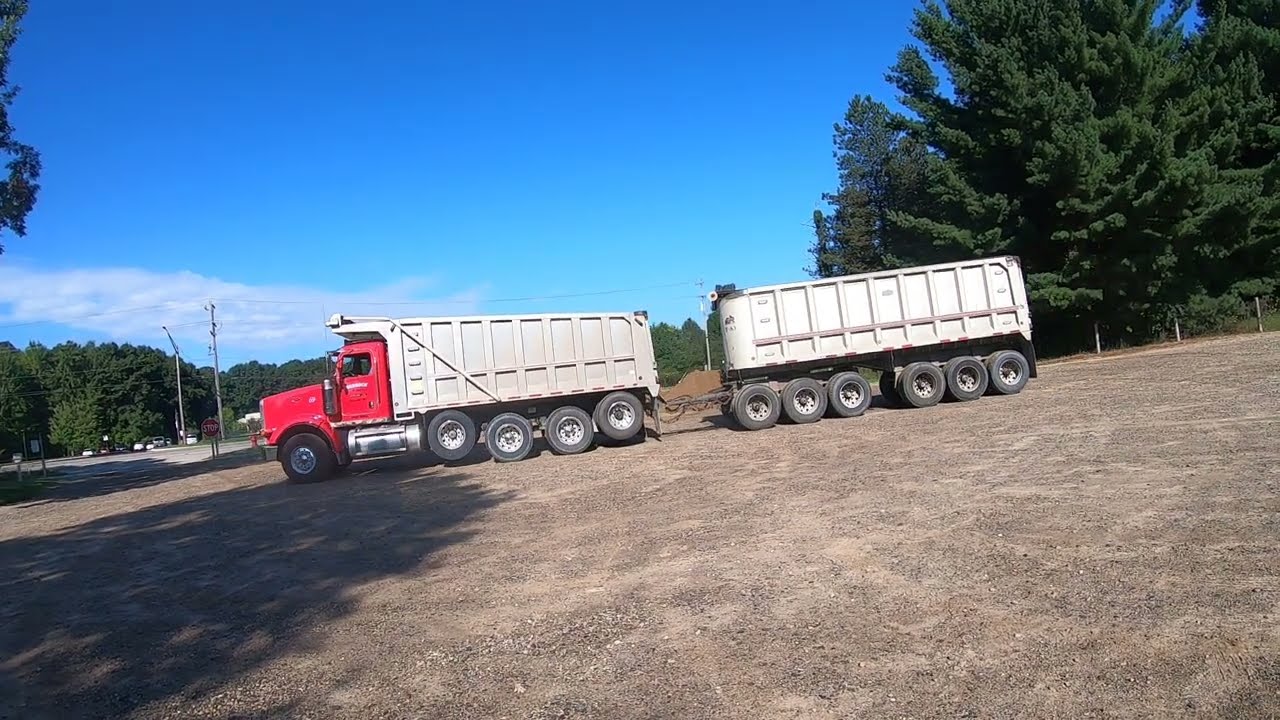The photograph features a long-haul truck with a bright red cab and a white trailer attached, showcasing a total of 11 visible wheels. The truck, resembling a Mack truck, is driving down a gravelly slope, headed towards a highway indicated by the presence of other vehicles and a stop sign in the distance. The clear blue sky, dotted with a few wisps of white clouds, serves as the backdrop. The scene is flanked by lush, green trees both in the foreground and scattered in the background, with a notably large, vibrant tree in the upper right corner. Utility poles can also be seen, adding to the outdoor, semi-industrial setting of the image.